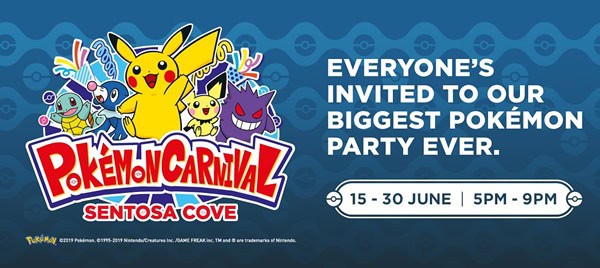This is a vibrant advertisement for the Pokémon Carnival at Sentosa Cove. The promotional poster features an inviting headline, "Everyone's invited to our biggest Pokémon party ever!", highlighting the event dates from June 15th to June 30th, 5 PM to 9 PM.

The background boasts a dark blue gradient that transitions from navy blue at the top to almost black at the bottom, embellished with subtle Pokéball graphics. Dominating the left side of the poster is a lively image of various Pokémon, with Pikachu taking center stage. Surrounding Pikachu are other fan favorites including Pichu, Squirtle, and Gengar, amid festive ribbons and party poppers.

The event title, "Pokémon Carnival Sentosa Cove", is prominently displayed in bold red font. Beneath this, in slightly smaller text, is the word "Pokémon", followed by even smaller font detailing the copyright and company name, though this text is difficult to discern.

This compelling advertisement sets the scene for an exciting Pokémon-themed celebration, sure to draw fans young and old.